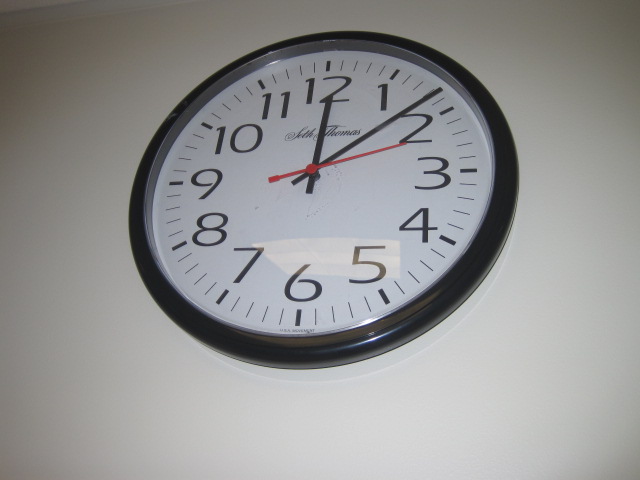This photograph features a circular wall clock, angled such that the viewer looks slightly upward at it, creating a subtle distortion. The clock, likely battery-powered, is encased in a black border with a white face. The numbers 1 through 12 are displayed in standard Arabic numerals in a black typeface. It features three hands: an hour hand, a minute hand, and a prominent bright red second hand. The time displayed is precisely 12:08 and 13 seconds. The brand name "Seth Thomas" is scripted elegantly just beneath the number 12. A plexiglass cover protects the clock face, reflecting a boxy, ceiling-mounted light fixture. The top edge of the photograph shows a small section where the wall meets the ceiling, further emphasizing the clock's likely placement on a white wall.